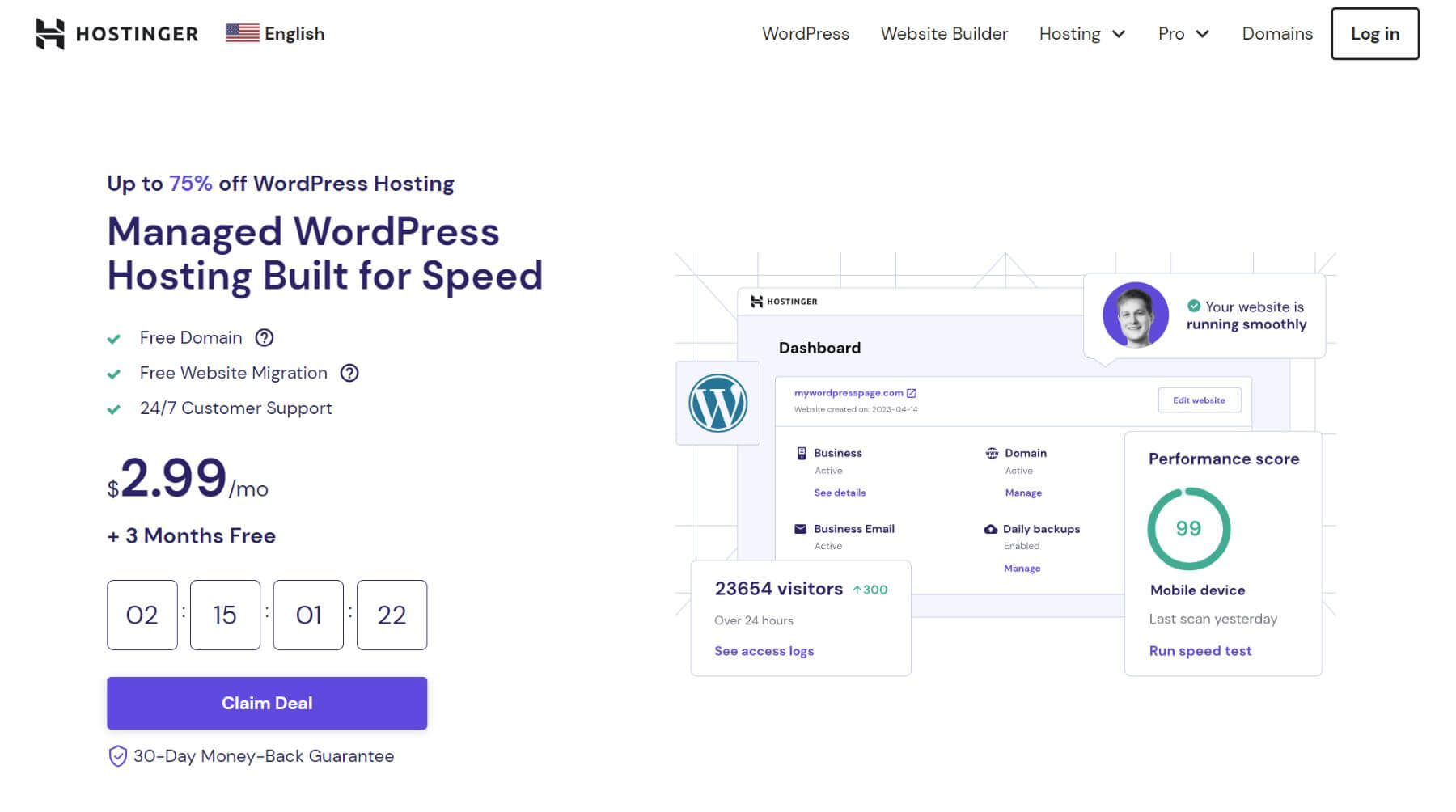**Caption:**

On the left-hand side against a white background, the header displays "Hostinger" in black next to an American flag, followed by "English." To the right, the navigation bar with black tabs reads "WordPress," "Website Builder," "Hosting," "Pro," and "Domains," with a black-bordered "Login" button beside it. 

On the left, a dark purple section offers a promotion: "Up to 75% off WordPress Hosting," with key features listed underneath marked by green check marks: "Free Domain," "Free Website Migration," "24/7 Customer Support." The pricing is highlighted as "$2.99/mo + 3 months free." Below, four outlined squares display "02," "15," "01," and "22," indicating specific metrics. A purple rectangle contains a white "Claim Deal" button, and below it, "30-day money-back guarantee" is mentioned.

On the right-hand side, in black text, it shows "Dashboard" and details the creation of a WordPress website on "2023-04-14." It states "Your website is running smoothly," with a performance score of "99" in green for mobile devices, last scanned "yesterday." Below, it shows "23654 visitors of 30000," highlighted in green.